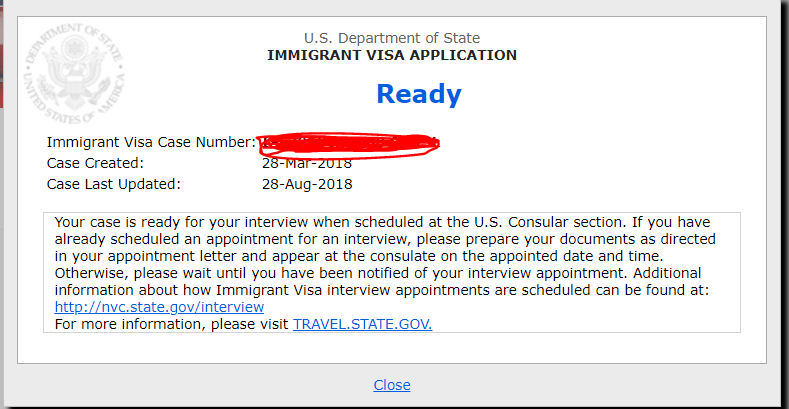The image depicts an online document from the U.S. Department of State regarding an immigration visa application. At the top center, the title "U.S. Department of State Immigration Visa Application" is prominently displayed. Directly below this title, the word "Ready" appears in a blue font. In the top left corner, there is a semi-transparent, light gray watermark featuring the official seal of the Department of State, with an eagle at its center.

The body of the document provides key details, including an "Immigrant Visa Case Number," though the case number itself is obscured by red ink. Further down, the document notes that the "Case Created" date is March 28, 2018, and the "Case Last Updated" date is August 28, 2018. The background of the document is plain white.

Throughout the document, there are three clickable links: one labeled "Closed" located at the very bottom, and two additional links to external websites. One of these links directs to a .gov site, while the other points to a State Department interview scheduling website.